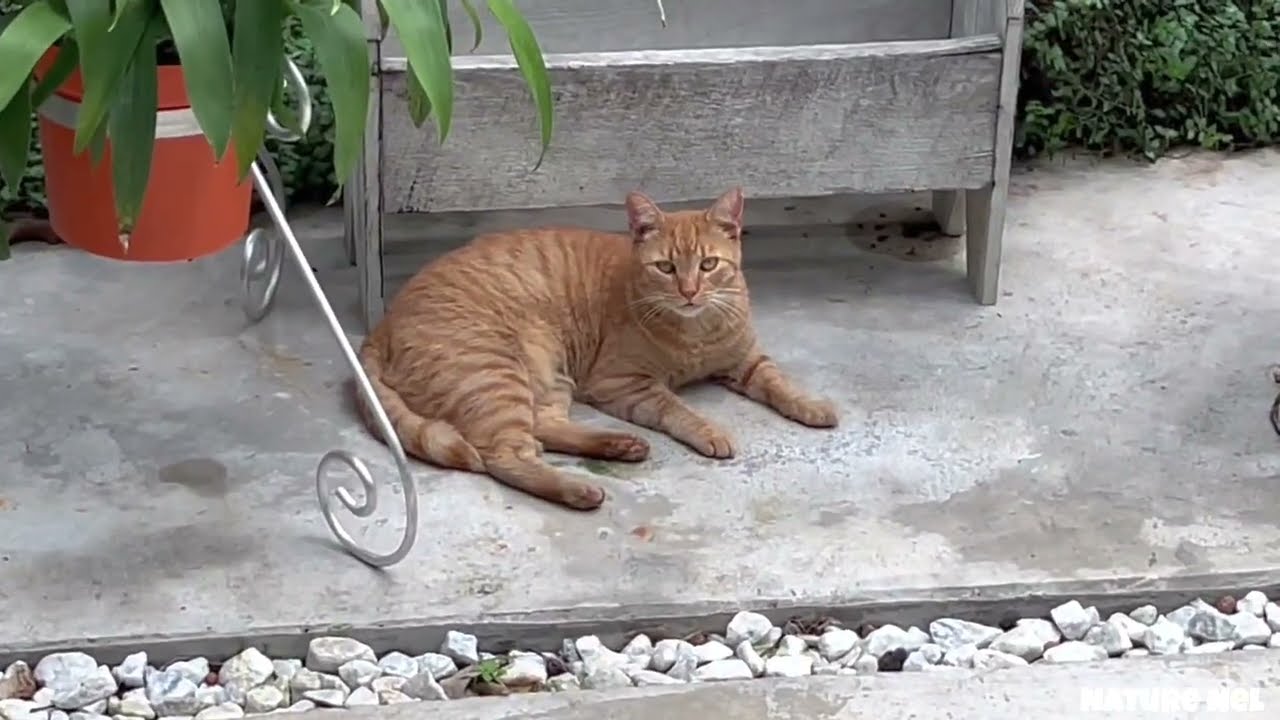In the image, we see an outdoor setting, perhaps someone's backyard, featuring an arrangement of various objects and a cat. Dominating the center of the image is an orange striped cat with yellow eyes and white whiskers, lying down on a light gray, slightly chipped and stained stone pavement. The cat is positioned horizontally with its head facing the right side of the frame and its tail towards the left, looking directly at the camera.

At the bottom of the picture, small rocks line the edge of the pavement, forming a gravel-filled drainage area. To the left of the cat, there is a scroll metal planter with intricately curled legs, which holds an orange-red pot with a white line around it; green leaves overflow from the pot. In the top left corner, there's another pot with plants.

In the background, on the back right corner, there is a silver, wood-topped bench next to some grass. Spanning the back of the image is a hedge of bushes, partially obscured by the wooden planter box situated behind the cat. The various colors present in the scene include green, orange, white, gray, tan, yellow, and red, suggesting it was taken outdoors in broad daylight.